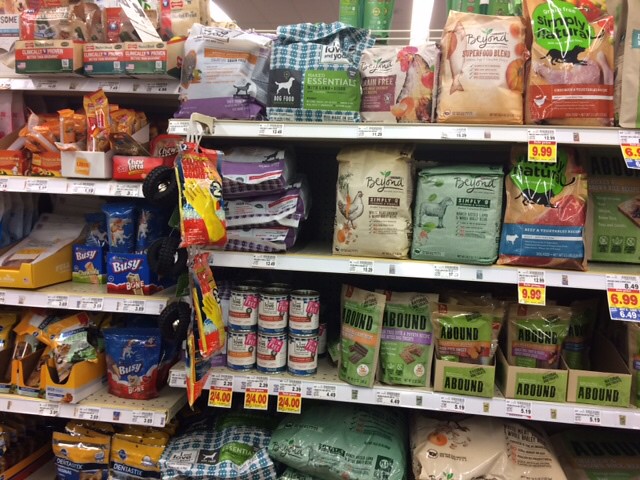This image showcases a grocery store shelf, likely from a Fry's Grocery Store, containing a variety of food and treats for pets, along with an impulse item for household chores. The top shelf on the right side displays bags of dog food, priced at $9.99 and $6.99, with some price tags partially out of view. The second shelf similarly holds bags of pet food, including ones labeled with images of a chicken and a lamb, possibly indicating different flavors. There is also a bag with a cat image, suggesting the presence of cat food. 

On the third shelf down, there are canned pet foods with a promotional price of two for four dollars. The bottom shelf holds large bags of dog food, with other treats visible on the left side of the image, including packages labeled "Busy." These 'Busy' products come in blue packaging with variations marked by green or red bottoms. Rubber dishwashing gloves in yellow packaging hang down from the shelves, positioned as impulse buy items. The price tags, characteristic of Fry's Grocery Store, mark some of the food items at $9.99, $6.99, and $24.